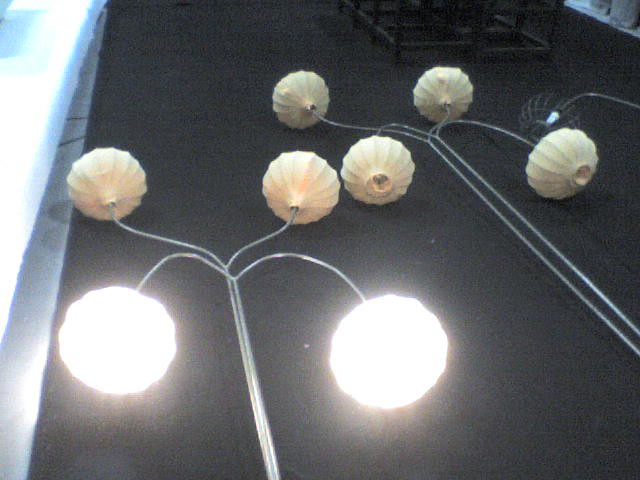This photograph features an intricate arrangement of silver lamps positioned on a black fabric surface, possibly a rug or table runner. The lamps have silver posts with branching metal lines that create a visually striking design. At the end of each branch, there are round, cream-colored lampshades with ridged edges, resembling seashells. Each post supports four lampshades. Specifically, two of the lampshades at the bottom left corner are illuminated, emitting bright white orbs of light, while the others remain turned off.

One lamp on the right appears as a separate fixture, characterized by an exposed wire and a pair of metal poles extending from its base. The lighting fixtures are arranged in a hooked and V-shaped manner, contributing to the unique aesthetic. In the background, a dark wooden table and a black metal structure can be faintly seen, subtly complementing the scene. The photograph effectively showcases the elegant design and varying lighting states of the fixtures, highlighting their potential ambiance when fully illuminated.